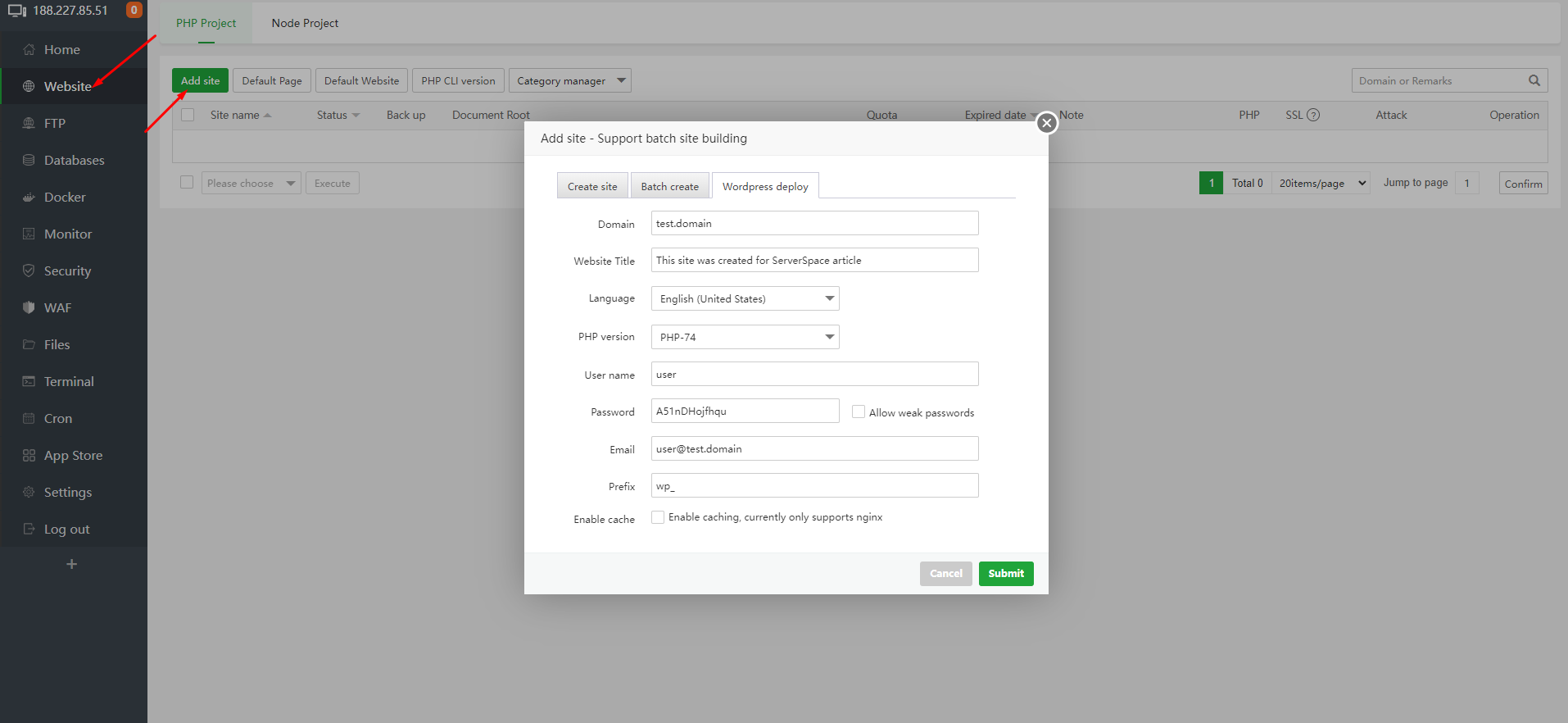In this image, we observe a detailed view of a web page interface. The interface comprises both a foreground and a background component. The foreground features a white dialog box, which seems to have been triggered by an interaction with the background. This foreground dialog box is titled "Add Site" and supports batch site creation. Within this dialog, there are three tabs labeled "Create Site," "Batch Create," and "WordPress Deploy."

The dialog box fields include options for "Domain," "Test Domain," "Website Title," "Language," "PHP Version," "Username," "Password," "Email," and "Prefix." Additionally, there are checkboxes for enabling cache and buttons for canceling or submitting this form, with the submit button being green.

In the background, the page includes a predominantly light gray or white interface with a vertical sidebar on the left, which is either black or navy blue. The sidebar lists several sections: "Home," "Website" (currently highlighted), "FTP," "Databases," "Docker," "Monitor," "Security," "WAF," "Files," "Terminal," "Cron," "App Store," "Settings," and "Logout." A plus icon is located below these options.

Dominating the right side of the background is a highlighted section showing a "PHP Project," followed by "Node Project," and an "Add Site" button. Below this, several other sections are visible, including "Default Page," "Default Website," "PHP CLI Version," and "Category Manager," showcasing various functionalities of the application.

Moreover, the image features direction indicators, with a red arrow pointing towards the highlighted "Website" section on the sidebar and another red arrow pointing towards the green "Add Site" button, guiding the user through key actionable items on the interface.